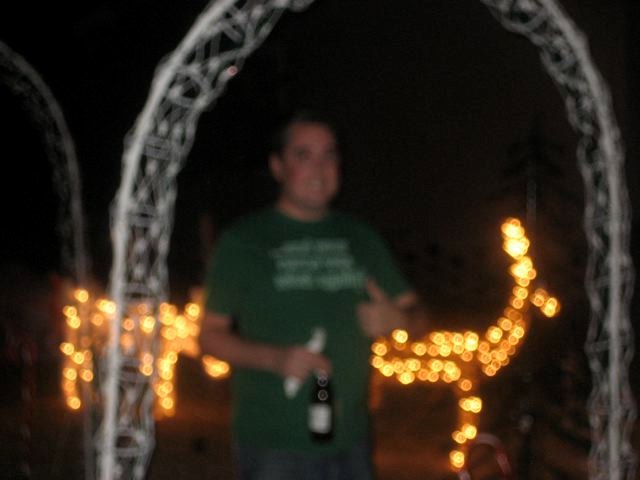A blurry nighttime photograph captures a man at what seems to be a festive celebration, possibly a Christmas-themed event. The focus of the camera is extremely close, rendering all distant details indistinct. The man wears a green t-shirt with unreadable white text and is smiling while giving a thumbs up with his left hand. In his right hand, he holds both a beer bottle and a white object. He stands under a thin white arch, likely part of a decorative Christmas tunnel. Behind him, two illuminated Christmas lawn deer with yellowish lights add a festive glow to the scene.